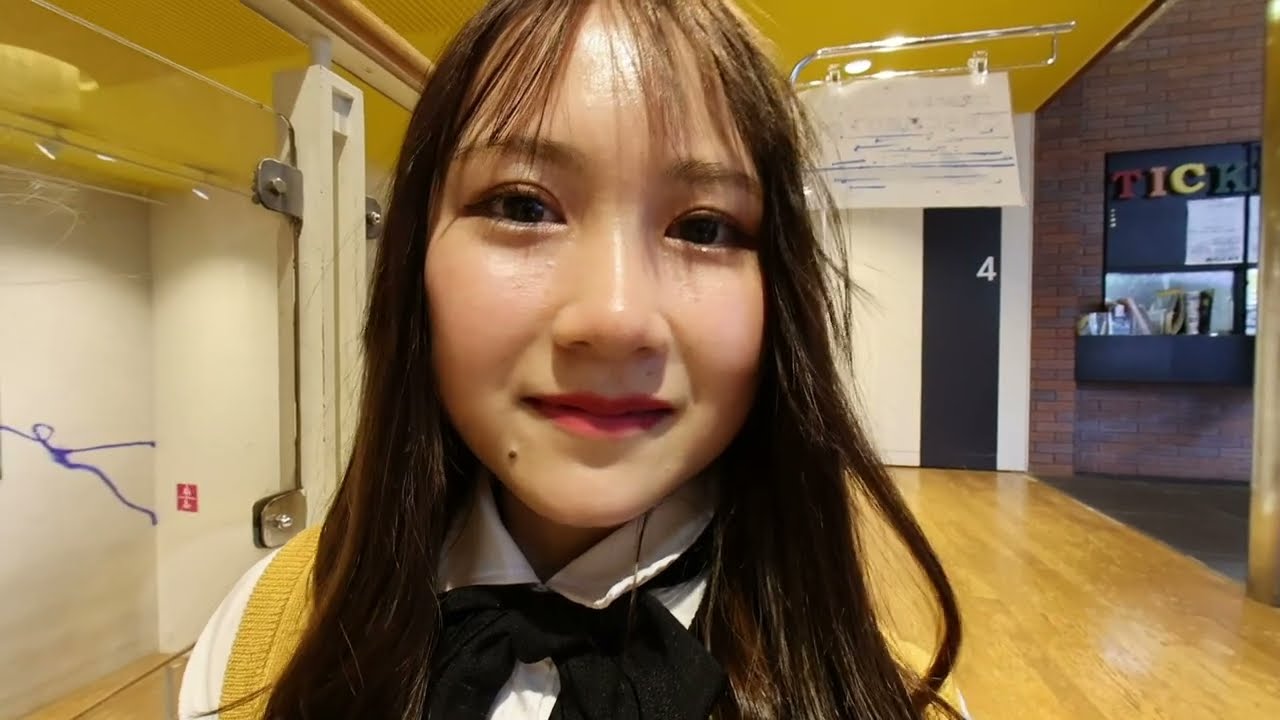A young Asian girl is capturing a close-up selfie, staring straight ahead with a mild, somewhat nervous smile. She has dark brown eyes, pink lips, and a small pimple just below her mouth on the left side. Her hair, with bangs almost touching her eyebrows, cascades past her shoulders and covers her ears. She is dressed in a white shirt with a black tie and a yellow vest, seemingly a uniform suggesting she might be working at a movie theater, as indicated by the letters "T-I-C-K" on a black display behind her—likely referring to 'tickets'. The backdrop features various elements: a shiny wooden floor, a black wall strip with a white number four, an opening revealing a brick wall, and a shelf with booklets and papers. The left side of the image displays a white wall streaked with purple graffiti, a red patch near its base, and predominantly yellow ceiling. The ambiance suggests a busy, potentially festive setting with party lights and graffiti, adding depth to the surrounding environment.